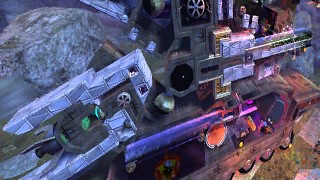The image features a backdrop of gray rocks adorned with patches of green, possibly indicating moss growth. Dominating the top-center of the picture are some metallic objects, while the bottom portion showcases machinery that resembles a saw or perhaps a tank with a series of wheels aligned in a row, mimicking tank treads. In the top-right corner, a metal piece that looks akin to a gun is visible, equipped with a rotating arm on its side. Intriguingly, there is a purple object situated in the middle of the scene.